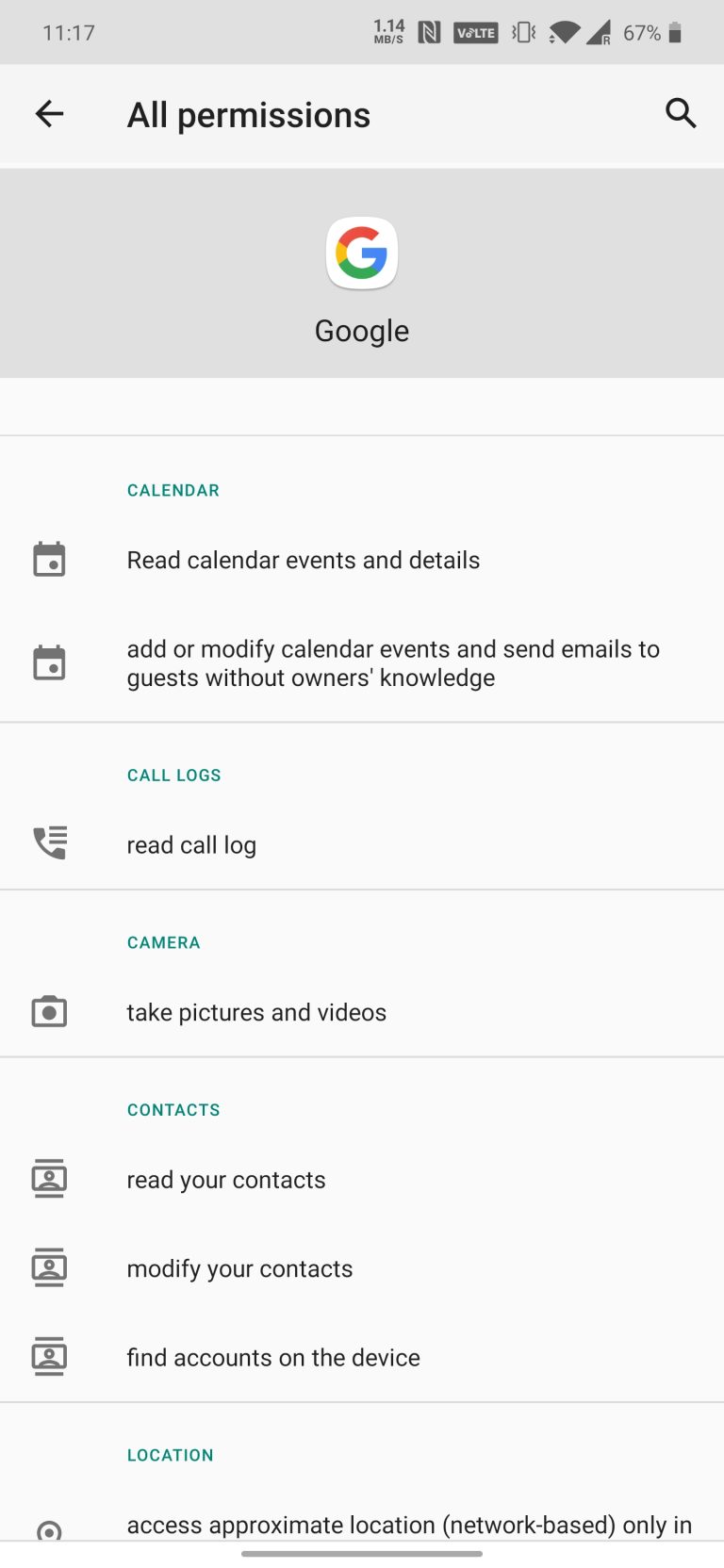The image depicts a screenshot of a cell phone permissions page. At the top, there is a light gray stripe displaying the time "11:17," a battery icon showing "67%," and signal indicators in small white squares. Below this, a lighter gray stripe features a left arrow labeled "All Permissions" and a search icon.

The main section consists of a large gray box with a Google logo, represented by a small square with red, yellow, green, and blue colors. This box is on a light gray background. Below the logo, in blue text, it says "Calendar," followed by a description in black text: "read calendar events and details, add or modify calendar events, and send emails to guests without the owner's knowledge."

Following a small dividing line, the next section highlights "Call Logs" in blue text, detailing "read call log" next to a small phone icon. Below that, the section for "Camera" in blue text states "take pictures and videos" in black.

Further down, "Contacts" in blue is followed by permissions listed in black: "read your contacts, modify your contacts, and find accounts on the device." The last section details location access, specifying "approximate location (network-based only)" above a gray dividing line.

Overall, the page outlines various permissions requested by Google, clearly categorized under separate headings for easy identification.